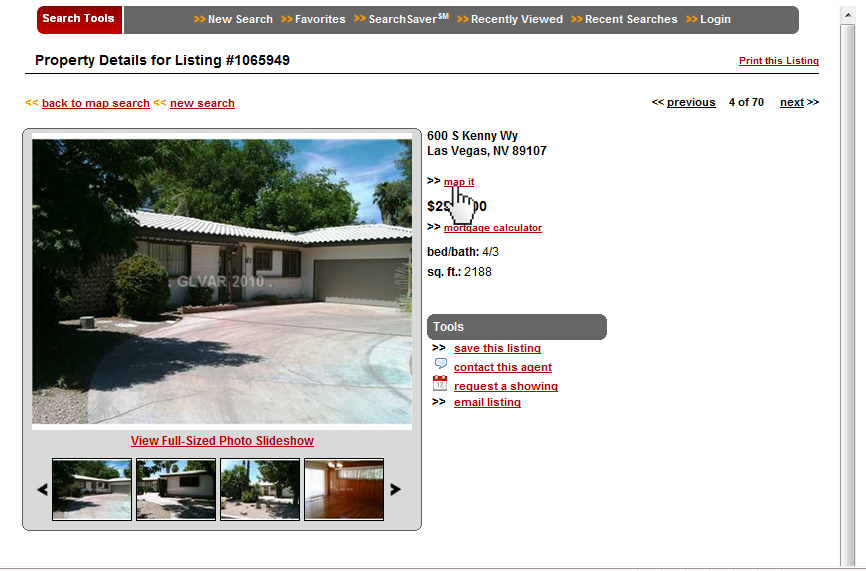This image is from a real estate listing for a property for sale in Las Vegas, Nevada, with listing number 1065949. The property is a single-story, white-painted house featuring long windows by the front door and a curved side leading to a two-car garage. The website interface shows navigation options, including "Search Tools," "New Search," "Favorites," "Search Saver," "Recently Viewed," "Recent Searches," and a "Log In" button at the top. The right-hand side displays a red, underlined "Print This Listing" link. The image also includes an area marked by a white hand cursor indicating "Map It." Further details provided include a four-bedroom, three-bathroom layout with a total living space of 2,188 square feet. Below the image, there are tools for a mortgage calculator and options to view a slideshow of full-size photos, revealing more visuals of the property.